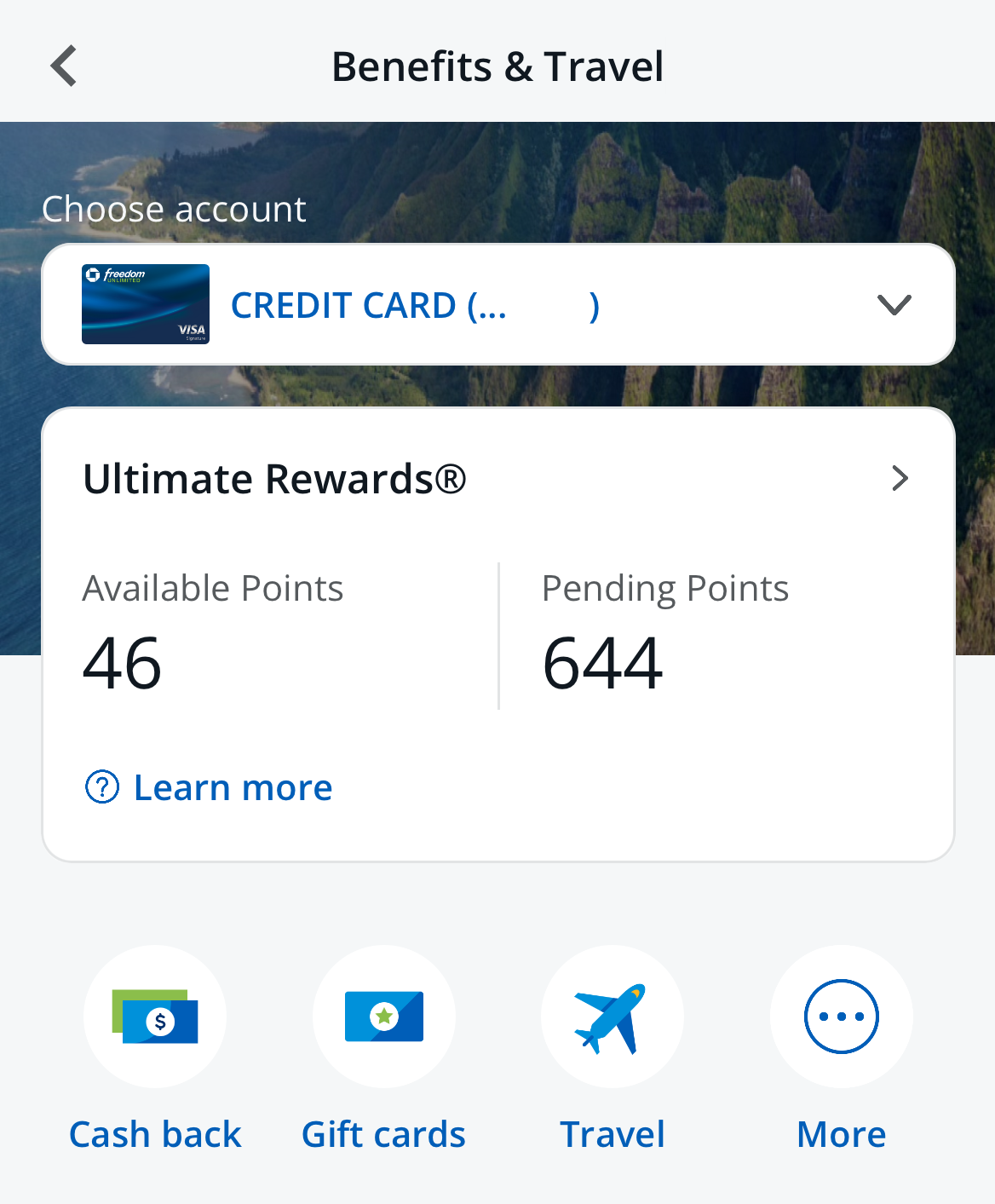The image appears to be a screenshot taken from a mobile device, such as a phone or tablet. At the top of the screen, there is a navigation bar featuring a left-facing arrow and the text "Benefits and Travel" in black font. Below this, the section labeled "Choose Account" is presented with an icon of a credit card and the text "Credit Card" in blue. An arrow pointing downward suggests additional options can be accessed. 

Further down, the "Ultimate Rewards" section displays available and pending points, specifically 46 available points and 644 pending points. A "Learn More" option is also visible. Below this section are icons arranged in a row, each representing different reward categories: 

1. "Cash Back" accompanied by an image of money.
2. "Gift Cards" symbolized with a card that has a star on it.
3. "Travel," indicated by a blue airplane icon.
4. "More," depicted with a circle containing three dots.

This detailed caption provides a comprehensive overview of each section and element within the image.